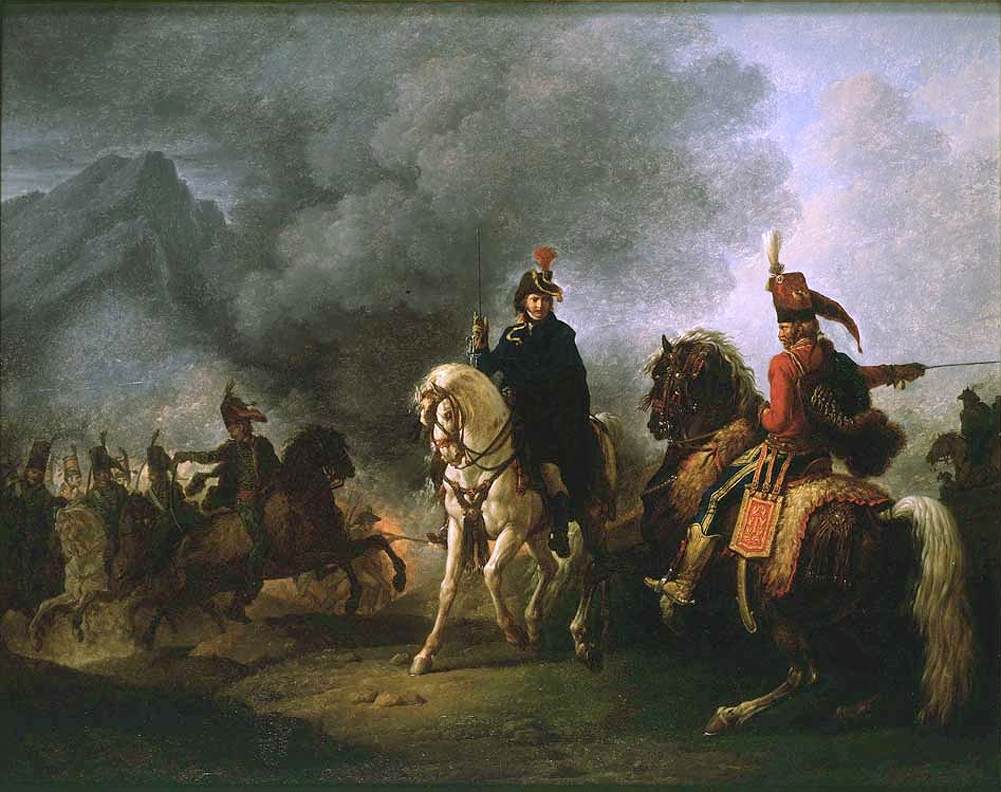This painting depicts a dramatic battlefield scene likely set between the 15th and 18th centuries. At the center, a commanding figure on a majestic white stallion raises his sword high, dressed in dark attire that includes a helmet with a distinctive tassel. Opposing him is another prominent figure on a sizeable brown stallion, adorned in a red jacket, blue pants, and gold boots, with a long red hat topped with white feathers. This man holds his sword and reins, appearing either in conversation or combat with the rider on the white horse. 

The background teems with activity, where a host of riders, resembling the central figure's attire, charge forward amidst billowing smoke that intermingles with the evening or nighttime sky. Hills loom in the distance, alongside indications of fire contributing to the smoke and creating an intense, chaotic scene. The battleground beneath the horses is strewn with stones and grass, painted in dark, earthen tones. This richly detailed scene, rife with historical military attire and action, captures the fervor and intensity of the era's warfare.